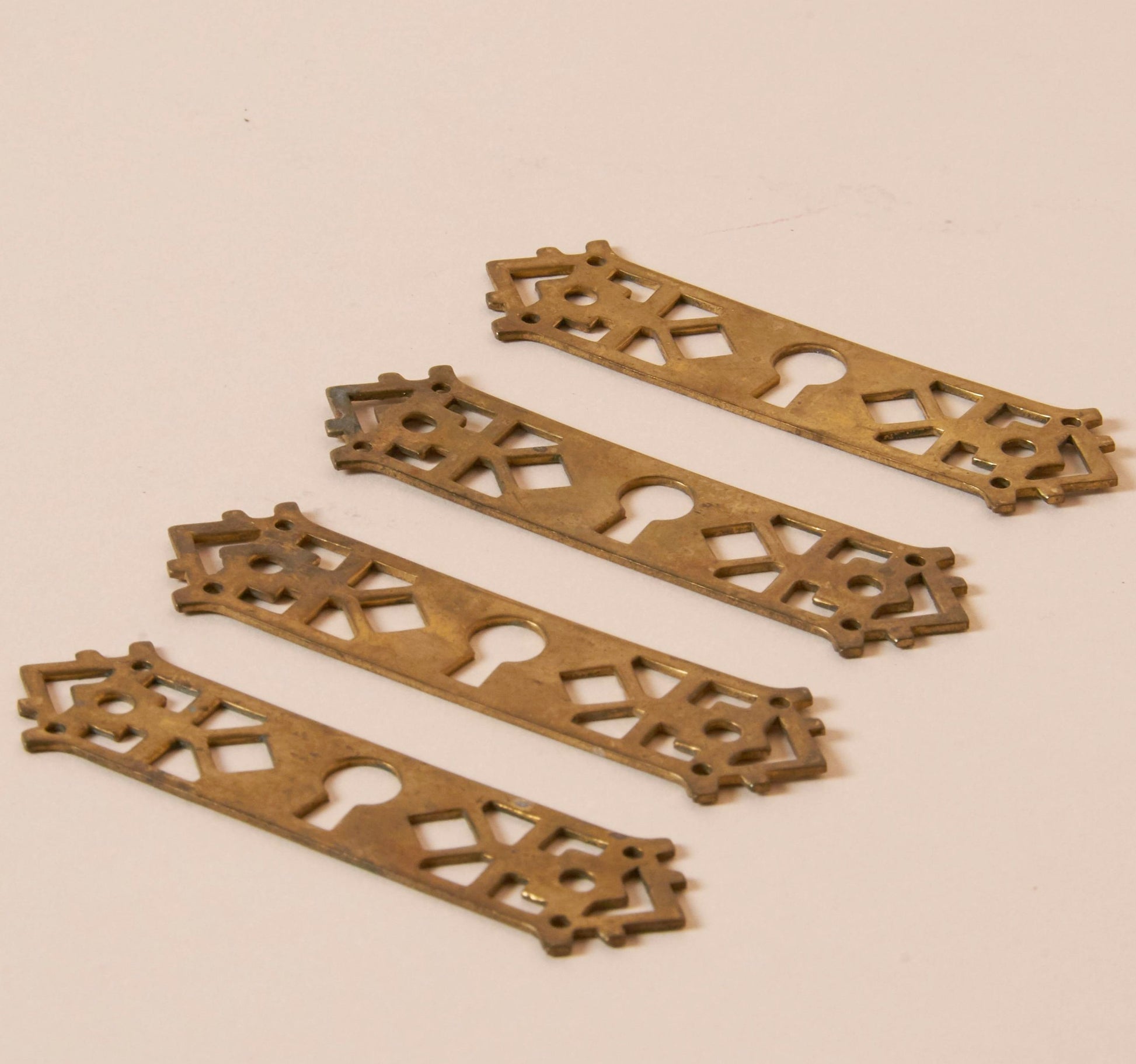This image features four identical escutcheon plates arranged diagonally from the bottom left to the top right against a peachy pink background. The plates appear to be made of a gold-toned brass, although they exhibit signs of age and distress, with blackened areas from oxidation. Each plate is designed with a central keyhole shape, evoking the form of an old-fashioned lock. The plates are ornamented with symmetrical patterns: two small triangles flanking a diamond, followed by the keyhole, and then mirrored on the opposite side. The edges of the plates are pointed or scalloped, enhancing their decorative appeal. With mounting holes on either side, these plates are likely meant for architectural use, perhaps to add vintage charm to furniture or doors. The overall composition suggests the image may be an advertisement for these decorative, antique-style pieces.